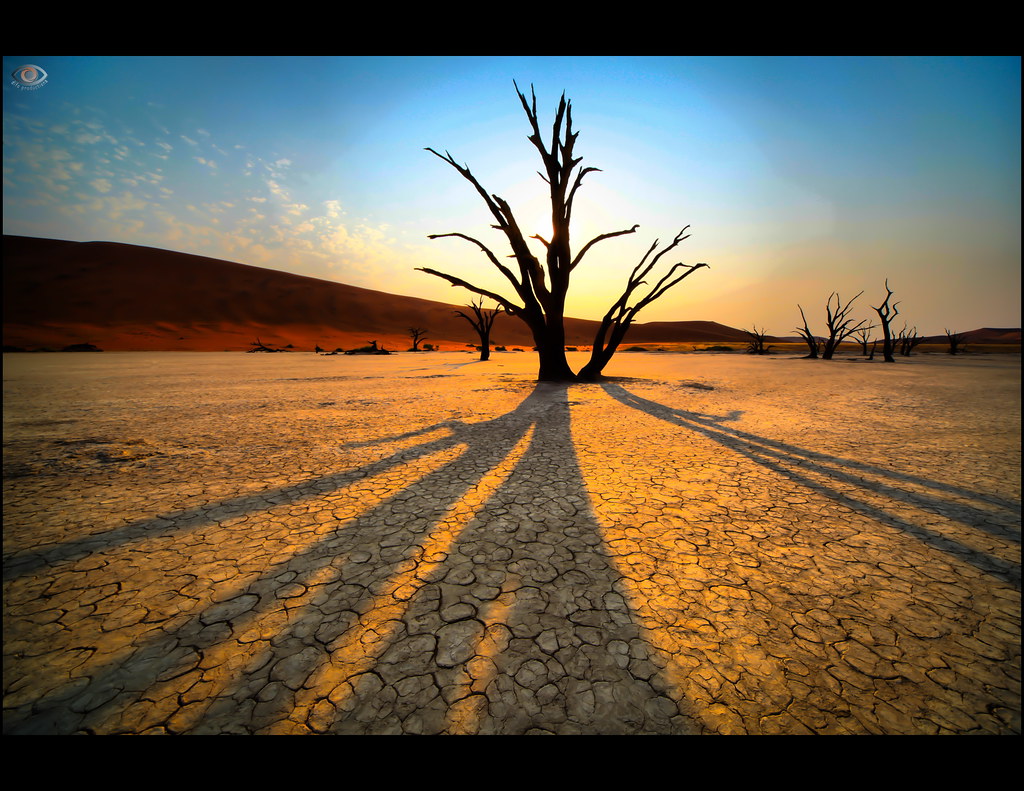A high-quality photograph captures a stark and arid desert scene bathed in daylight under a clear blue sky with scattered puffy clouds to the left. Dominating the foreground, the cracked, light brown, and parched ground reflects the harshness of the environment. Prominently positioned in the center is a bare, leafless tree casting a long, well-defined shadow stretching towards the camera, highlighting the texture of the cracked earth beneath. In the background, dark brown or black skeletal trees with extensive branching suggest a landscape marked by desolation, perhaps due to disease or extreme dryness. To the left and trailing into the background, the terrain transitions into rolling desert hills of lighter and darker brown shades, while a subtle hint of a sunset adds a warm yellow hue to the scene. At the top and bottom of the image, black bars frame the photograph, with a small eye logo situated in the top left corner.